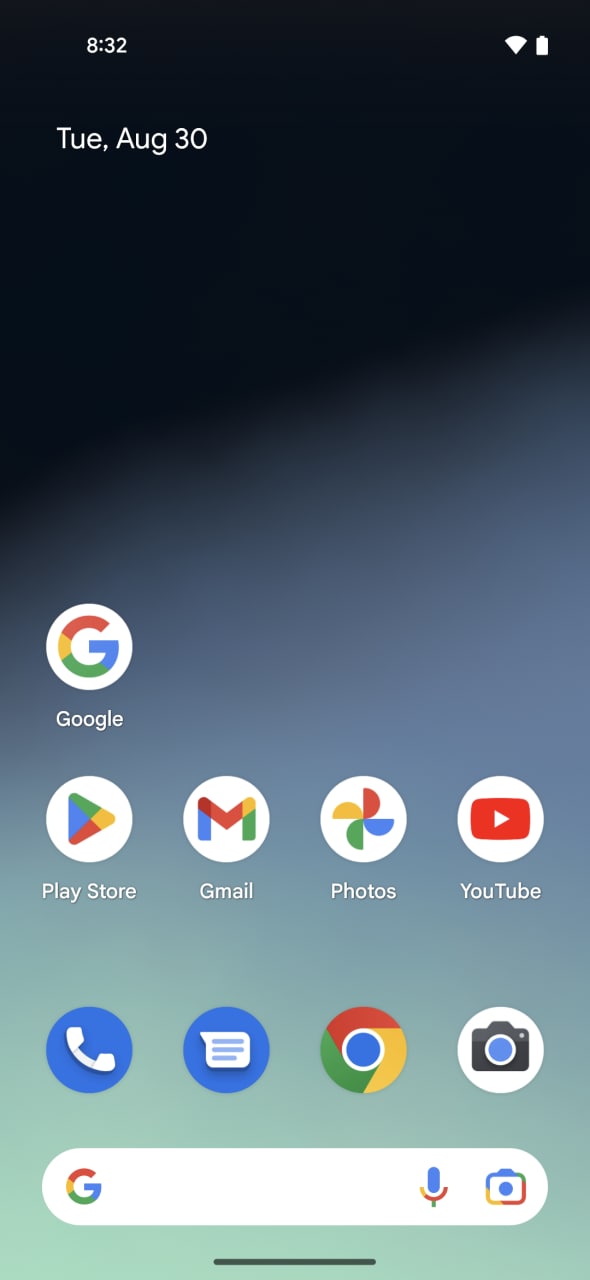A digital screenshot showing the home screen of a smartphone displays a variety of visual elements. The current time, 8:32, is prominently positioned at the top of the screen, accompanied by full and white Wi-Fi and battery icons to the right. Directly beneath the time is the date, which reads "Tuesday, August 30th."

Occupying the main portion of the screenshot are various app icons. Notable among these is the Google app, featuring a logo comprised of the colors red, yellow, green, and blue. The Play Store icon is also visible, characterized by a sideways triangular shape in red, green, and yellow.

Other app icons include Gmail, identified by its distinctive 'M' in blue, red, yellow, and green. The Photos app and the YouTube app are present as well, with the latter featuring a red play button set against a yellow and red backdrop. Additionally, there is a camera app, depicted by an image of a camera, and the Google Chrome app. Lastly, a phone app and a search bar are visible on the screen.